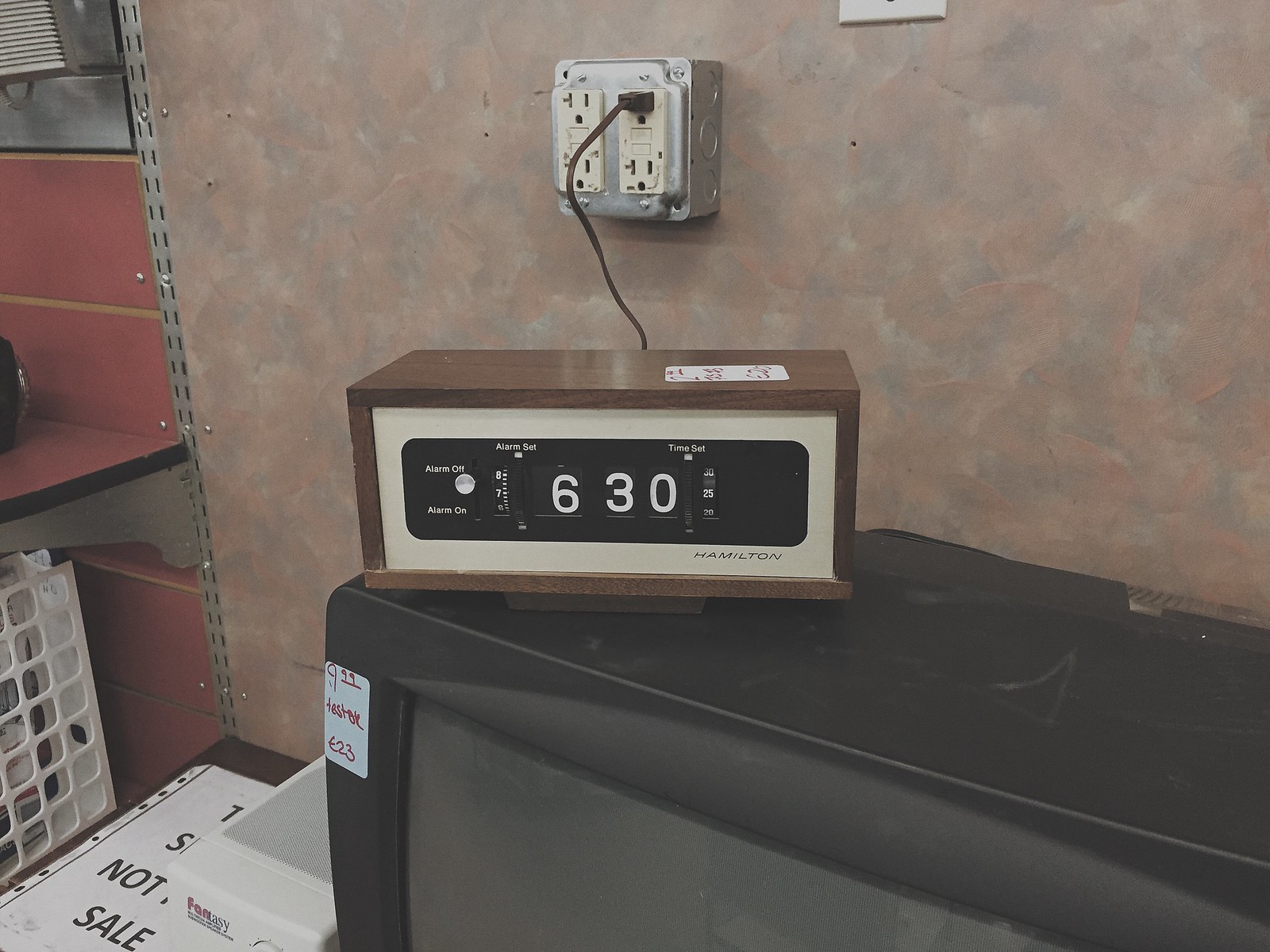In this image, we see an old-fashioned alarm clock with a wood finish and a cream-colored insert, featuring flip numbers to display the time, which reads 6:30. The clock, resembling a radio clock with various controls labeled "alarm off" and "alarm on," sits atop a black, boxy television set. A handwritten price tag on the clock indicates it is for sale at $9.99, likely in a second-hand store. The clock is plugged into a brown-colored wall outlet with four sockets, utilizing the top right plug. The background also features red shelves on the left, a white basket organizer, and part of a sign that says "not for sale." The scene is characterized by a nostalgic ambiance, emphasized by the overall older appearance and the use of filters, possibly suggesting it was taken with an older camera.